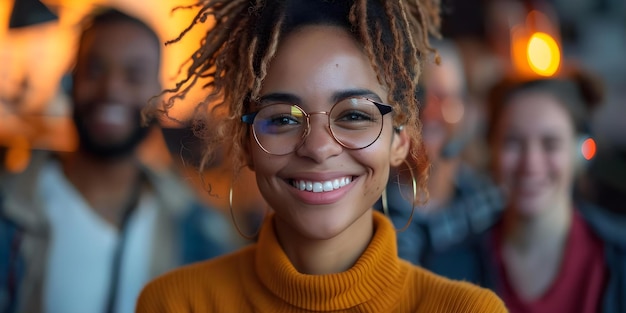A vibrant young African-American woman is the focal point of this photograph, her joyful smile radiating warmth. She is in her 20s, wearing a stylish orange turtleneck sweater, though the image is cropped just above her shoulders. Her hair, styled in voluminous dreadlocks, frames her face beautifully as it cascades down from the center of her head. She dons round wire-rimmed glasses that add a touch of intellectual charm. In the blurred background, an African-American man stands slightly to her left, while to her right, another woman, whose ethnicity is indistinguishable, completes the scene. The overall composition highlights the woman’s exuberant essence, captured in a moment of genuine happiness.